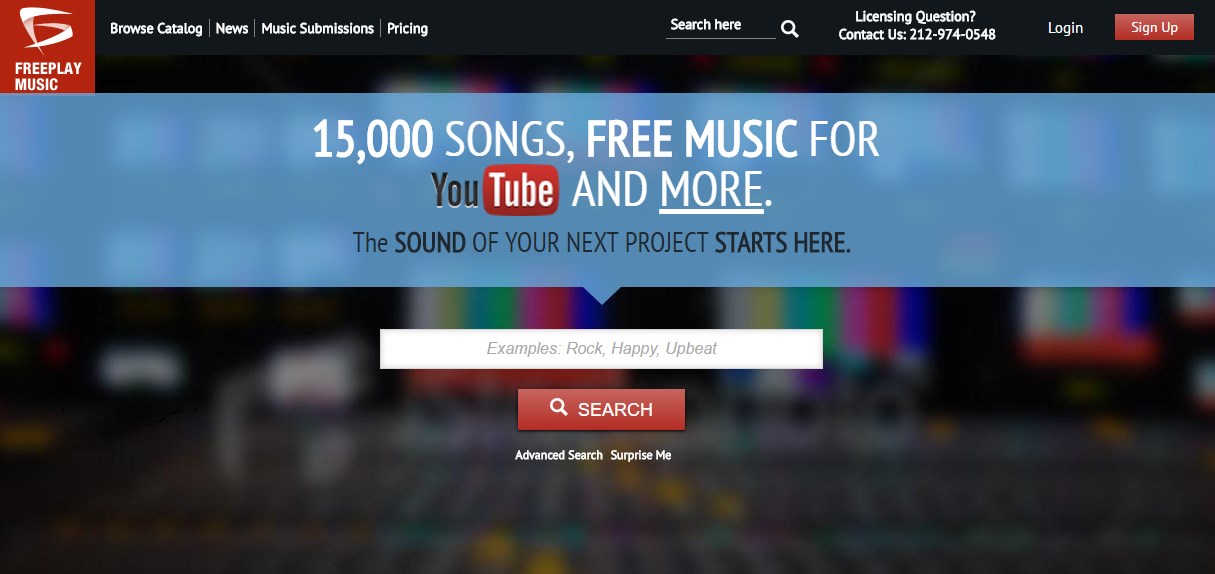The image is a widescreen snapshot of a website titled "FreePlay Music," as indicated in the top left-hand corner. Adjacent to the title, the website's navigation links—Browse, Catalog, News, Music Submissions, and Pricing—are displayed in white text against a black background. The main content area features a blurry backdrop that resembles a studio environment. Prominently centered in the foreground is a bold white headline proclaiming "15,000 songs, free music for YouTube and more." Below this headline is a red search button labeled "Search" in white text, adjacent to a search bar that provides example search terms such as "Rock," "Happy," and "Upbeat." Additional options for "Advanced Search" and "Surprise Me" are positioned beneath the search bar. In the top right-hand corner, users can find options to log in or sign up, along with a "Contact Us" number. Another search bar is located at the top center of the page, completing the functional and navigational elements of the website's design.